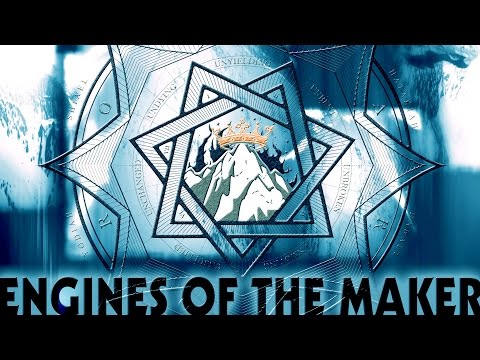The image appears to be a promotional poster or album cover with distinctive black borders at the top and bottom. Dominating the center of the image is a meticulously designed logo. This logo features a mountain covered in white and gray hues with a gold crown perched on its peak, symbolizing majesty or leadership. Surrounding the mountain, there are overlapping shapes: two square borders intersected to form a seven-pointed star, encased within a larger star, all of which is placed inside a circle. The backdrop of this intricate design has an ice-like texture, enhancing the visual complexity.

Supporting the central imagery, the background displays a mix of dark greenish-blue and white areas on the sides, adding depth and contrast. Encompassing the seven-pointed star are the words "undying, unyielding, unbroken" in light gray text, emphasizing themes of resilience and strength.

At the bottom, just above the black border, the phrase "Engines of the Maker" is prominently displayed in bold, black font, anchoring the image and providing a title that hints at creation or innovation. The overall color scheme of the poster is dominated by various shades of blue, tying all the elements together into a cohesive and striking visual presentation.